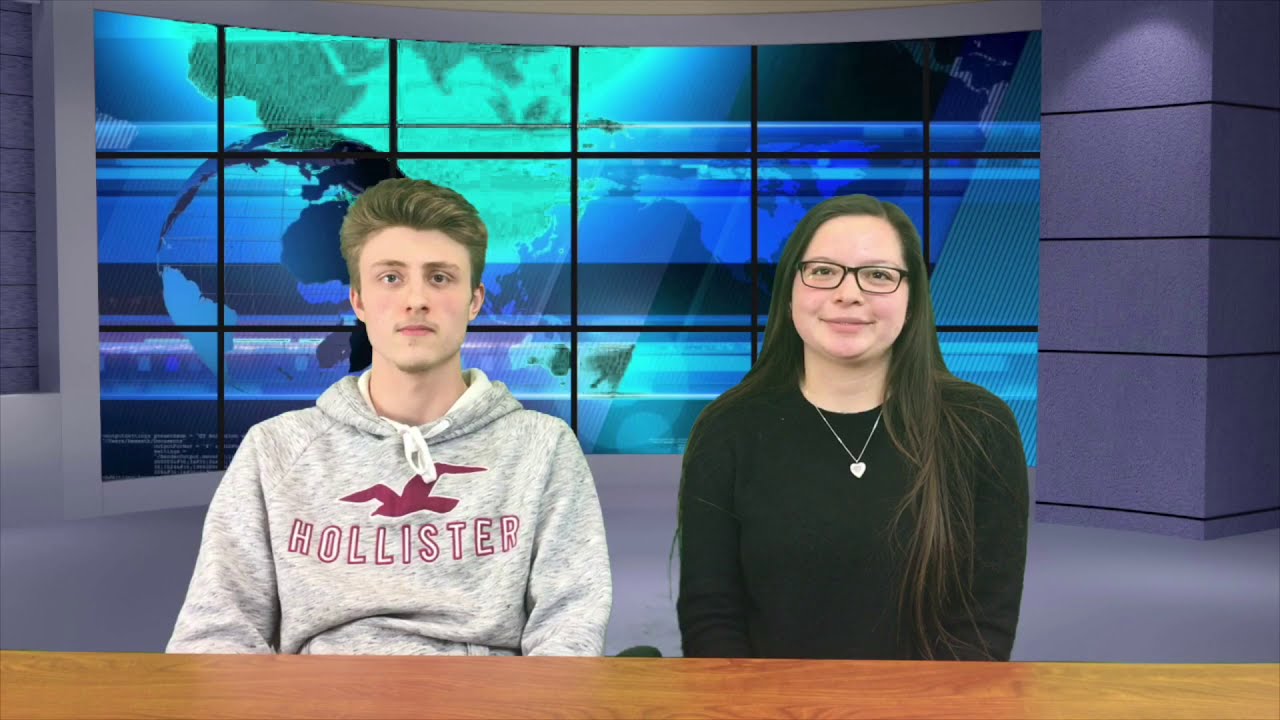In this image, we see a young Caucasian man and woman, who appear to be news anchors, sitting at a plain wooden desk, likely engaged in a student news broadcast. The man is on the left side, sporting short, light brown hair styled upwards, a thin blonde mustache, and a hint of stubble on his chin. He is dressed in a gray hooded sweatshirt with "Hollister" embossed in red block letters and a burgundy seagull logo above it. To his right sits a woman with long brown hair cascading down to her stomach, wearing black glasses, a black long-sleeved sweater, and a silver chain necklace featuring a small heart pendant. A curved, purplish-blue backdrop envelops them, adorned with a large video screen showcasing a 3D globe on the left, surrounded by green continents against a blue background filled with outlined continents and various patterns. Both of them face forward, with the woman smiling slightly and the man maintaining a neutral expression.